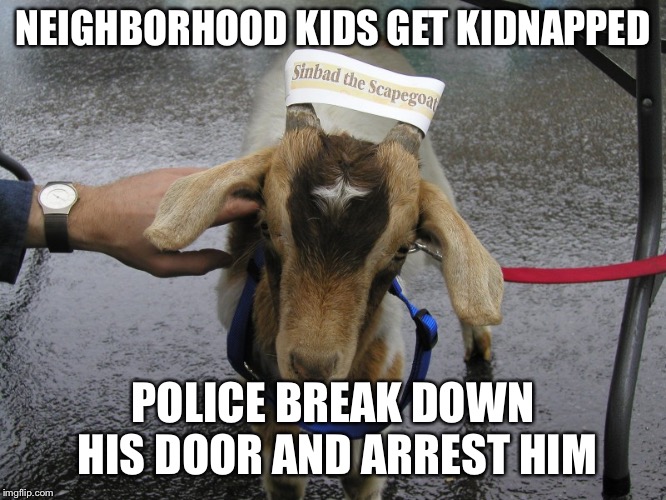The image is a detailed meme photograph featuring a small goat at the center, with light brown fur and a distinctive darker brown spot on its forehead that has a white patch in the center. The goat has two gray horns with a white piece of paper wrapped around them, bearing the text "Sinbad the scapegoat" in black letters. The goat is outfitted with a blue harness to which a red leash is attached. A human hand, presumably male, is visible on the left side of the image, petting the goat's head. This hand is wearing a black watch with a white face. The background shows a dark, rainy, and wet cement surface. Overlaying the top of the photograph in large, all-caps white text with a black border, is the caption "NEIGHBORHOOD KIDS GET KIDNAPPED." Similarly, at the bottom of the image, in two rows of the same style text, it reads "POLICE BREAK DOWN HIS DOOR AND ARREST HIM." At the bottom left corner, an extremely small white text watermark reads "imgflip.com."